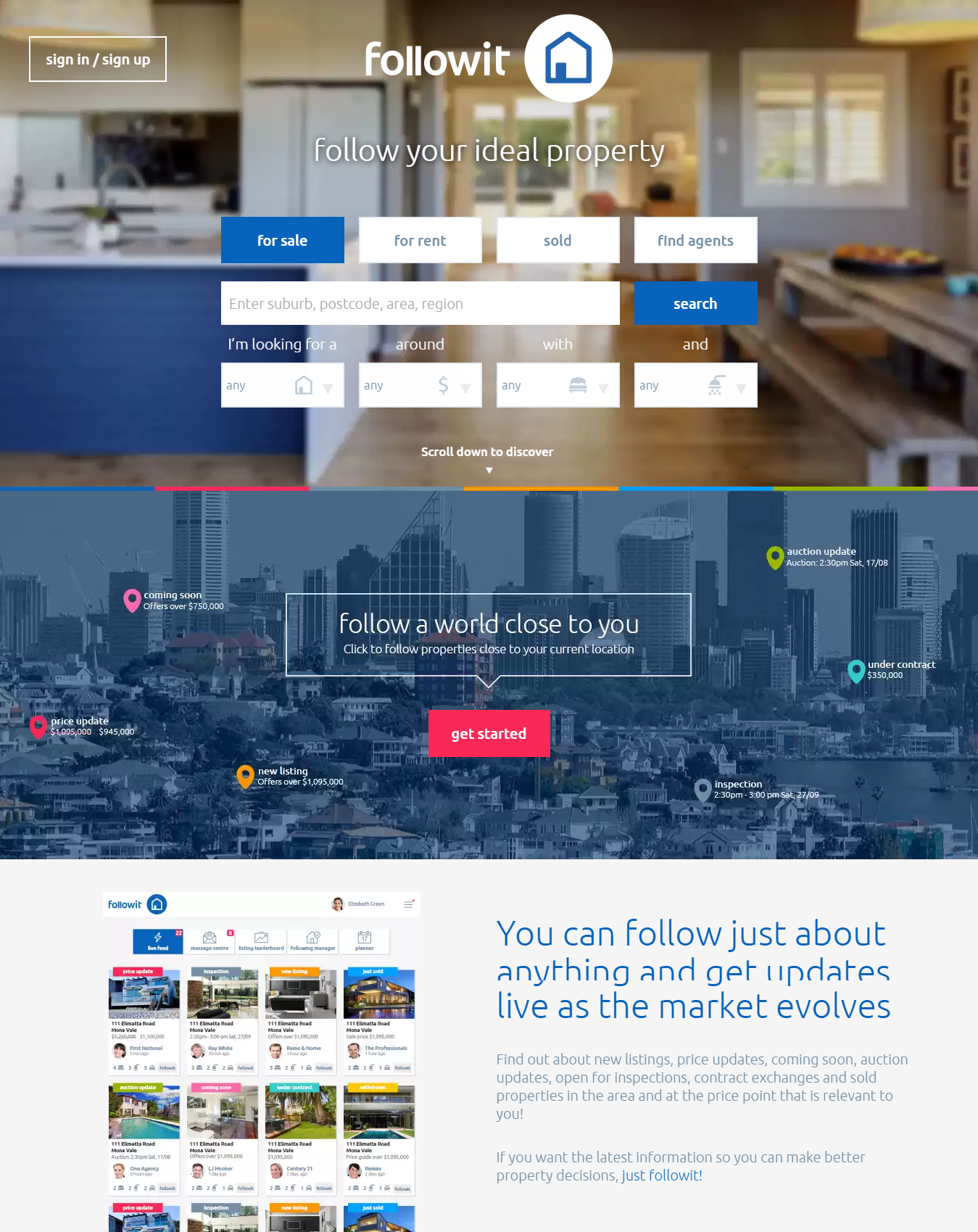This screenshot captures a webpage featuring a vibrant kitchen scene at the top. The image showcases a kitchen with a rustic appeal, highlighted by a hardwood floor. On the right, there's a rough-hewn wooden picnic table with a built-in bench, while a kitchen island stands to the left. This island is striking with its blue base and white countertop, featuring a prominent sink faucet. A white refrigerator is visible amidst the natural light flooding the space, suggesting that no artificial lights are on.

Superimposed on the upper left corner of this image is a white-outlined rectangle with the text "Sign In / Sign Up" in white font. At the center top, "Follow Wit" appears in similar white font, accompanied by a white circle bearing a blue house icon, and the phrase "Follow Your Ideal Property" beneath it. Below this, four small rectangles serve as navigation tabs: the far left one is blue with "For Sale" in white font, while the other three are white with black text reading "For Rent," "Sold," and "Find Agents," respectively. 

Toward the bottom of the screenshot, a search field prompts users with the gray-text instruction: "Enter suburb, postcode, area, region."